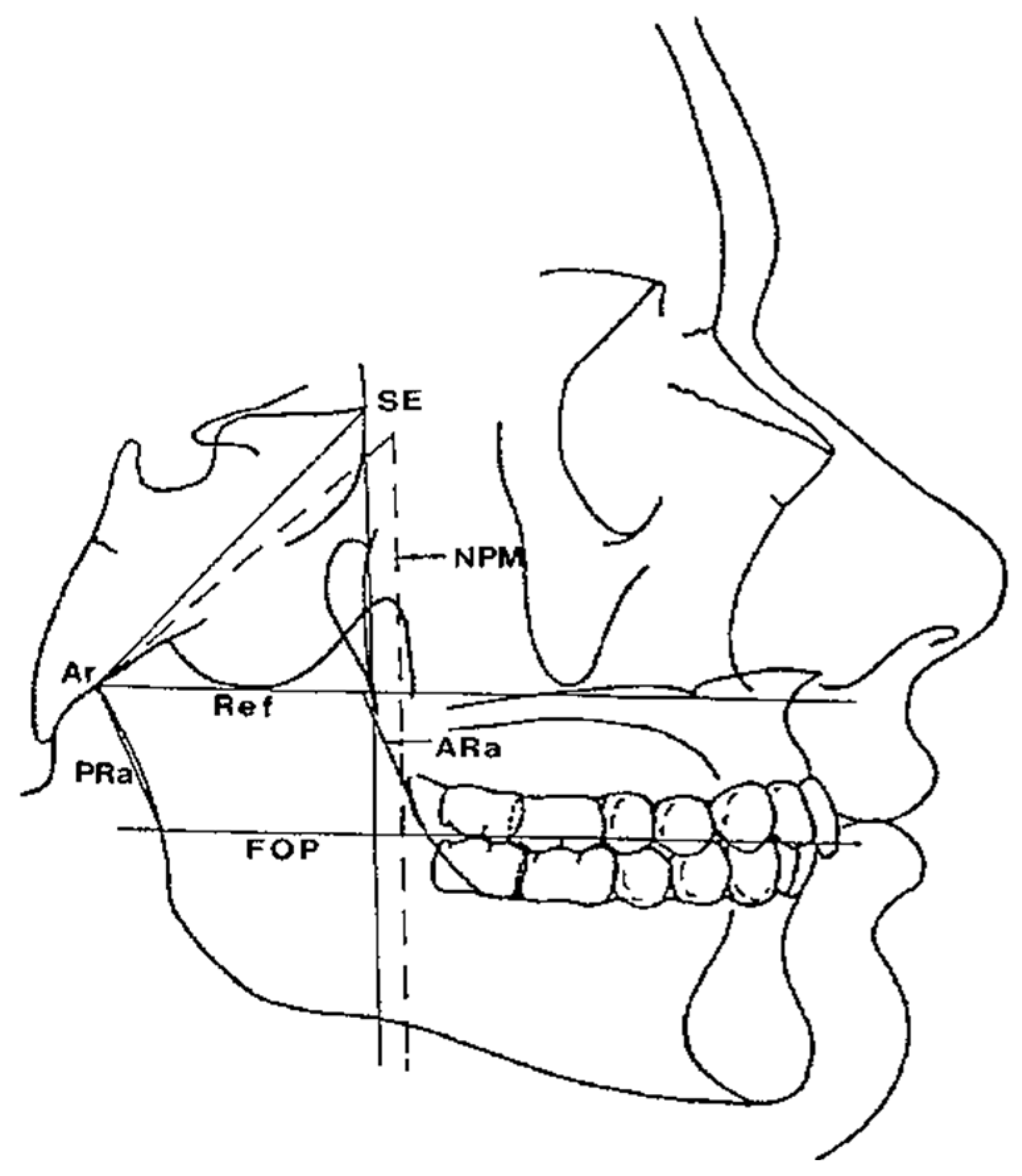This is a detailed black and white medical line drawing depicting a profile view of a human head, facing right. The illustration, outlined in black against a plain white background, features both the flesh profile and the underlying skull structure. From the forehead, it follows the contour down through the nose, lips, and chin, while the back of the head extends from the skull base, connecting to the chin.

The image includes intricate details such as a curved line representing the right nostril and another for the closed lips, with the teeth illustrated inside the mouth. The skeletal structure highlights visible bone features like the eye socket, nasal cavity, and jawbone.

Several lines are also present: a horizontal line through the center of the teeth marked "FOP," another horizontal line above it labeled "REF," and a solid vertical line behind the teeth denoted as "SE" with a dashed vertical line in front of it labeled "NPM." Additionally, the skull features labels such as "AR" and "PRA" toward the left side, and "ARA" on the jawbone.